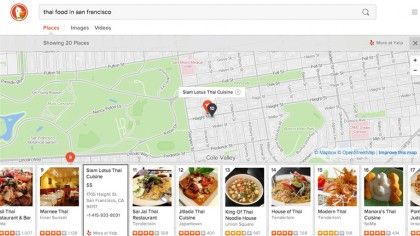This is a screenshot of a DuckDuckGo search results page. At the top left corner, the DuckDuckGo logo featuring the iconic duck is clearly visible, adjacent to the search bar. The search query typed into the bar reads "thai food in san francisco" in lowercase letters. Beneath the search bar are three tabs labeled "Places," "Images," and "Videos." The "Places" tab is highlighted in orange, indicating it is currently selected, while the other two tabs remain gray.

Directly below the tabs, there is a small orange triangle pointing upwards towards the "Places" tab with the text "Showing 20 places" beneath it. Following this, a partial map of a neighborhood is displayed, marked with pins that signify various locations offering Thai food. However, due to the blurriness of the image, the names of these locations are difficult to discern.

Scrolling further down, there is a list of different Thai food establishments. Each entry comprises a small numbered triangle at the top left corner, an image depicting either the food or the restaurant interior, the name of the restaurant, and beneath that, the corresponding Yelp star ratings. Despite the overall blurriness, the layout and essential elements of the search results can still be identified.